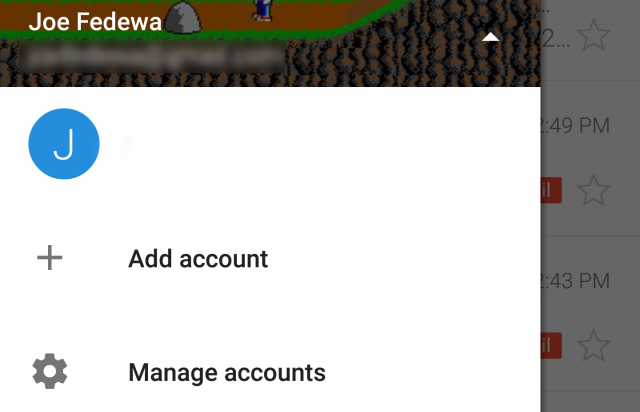The image features a multicolored background. At the top, there's a brownish section with "Joe Fedewa" written in white text. Below this, the background transitions to brown, and you can see part of a character's legs clad in blue pants and a white jacket. A thin green line separates this section from a gray one beneath it. 

In the gray area, there's a white upward arrow pointing towards a light gray paper icon to the side. Adjacent to these icons, you can see a time stamp of "1:49 PM" accompanied by a star and a number "2". Towards the right, there's a small orange box with another star and a time stamp of "4:43 PM," followed by an additional orange box and star.

At the bottom, a white box appears, overlaying other elements. Inside this box, there's a prominent blue circle with a white "J" in its center. Next to this circle, there's a plus sign and the text "Add account." A cog icon labeled "Manage accounts" is also present in black print. This scene is part of the user interface for a site associated with "Joe Fedewa," marked notably by the blue circle with the "J," the option to "Add account," and the "Manage accounts" settings.